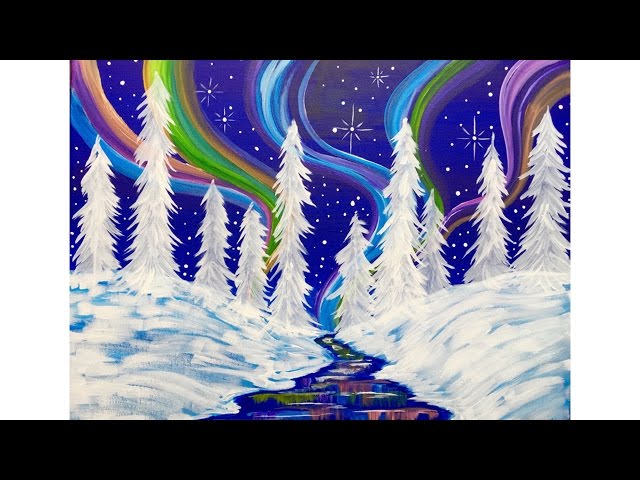This captivating digital illustration portrays a serene winterscape imbued with whimsical fantasy elements. Dominating the scene is a small, deep blue creek that gently meanders between snow-covered banks. Along these banks stand ten tall, slender pine trees, their branches laden with pristine white snow, enhancing the sense of frozen tranquility. The sky above is a canvas of vibrant artistry, adorned with five colorful swirls—blue, purple, green, yellow, and orange—that resemble the majestic northern lights. These multicolored streaks paint the sky with an otherworldly glow, mirrored beautifully in the water below. Adding to the magical ambiance, the sky is also sprinkled with numerous bright white stars, giving the impression of a festive, almost Christmas-like atmosphere.